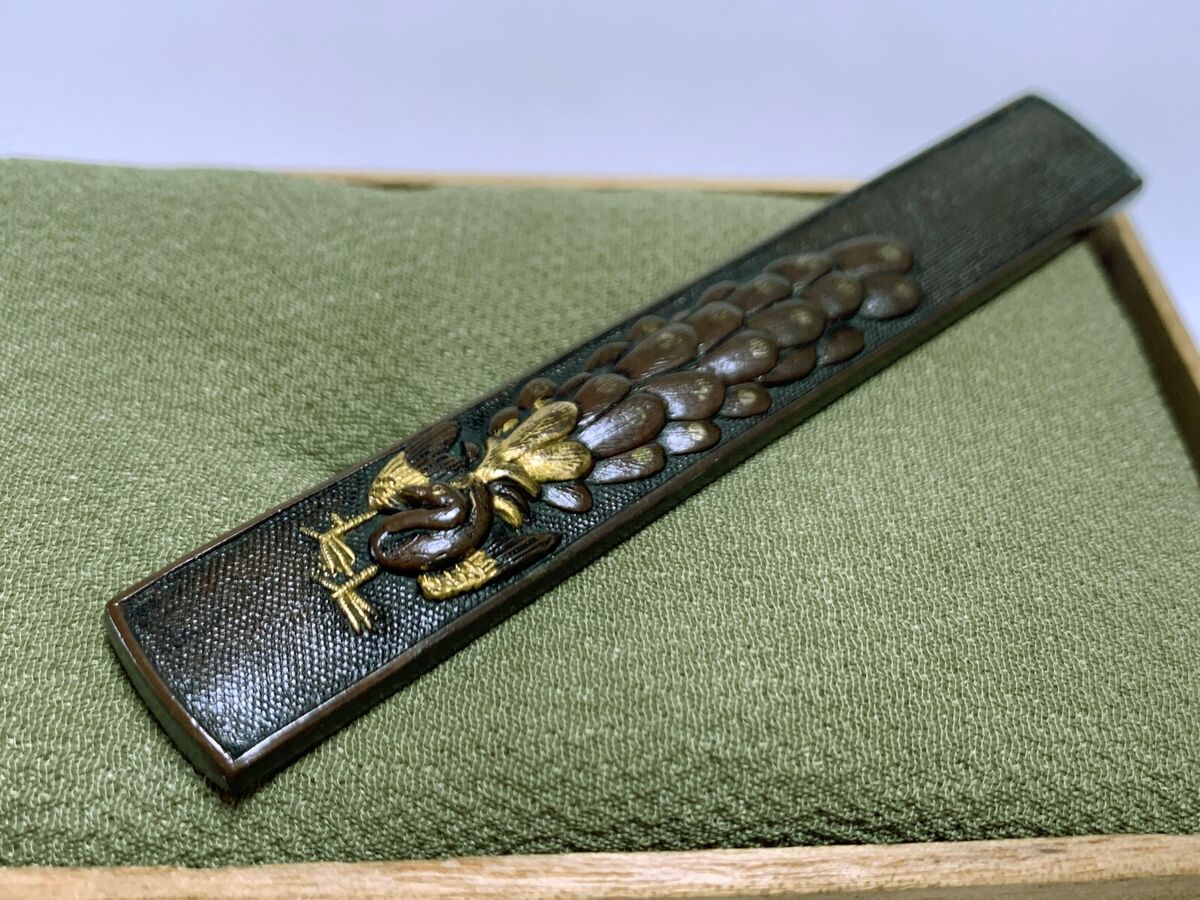This is a detailed photograph featuring a rectangular sheath designed for holding a sword, lying on a green footstool-like surface, upholstered with green fabric. The background features a blue wall. The sheath itself showcases intricate artwork of a bird, possibly a large turkey. The bird is predominantly brown with golden wings, legs, and plumes on its head, though the tips of the wings and the extended plumes transition to brown. The sheath is primarily dark brown but has lighter brown accents similar to the bird's feathers, offering a subtle contrast. The overall setting gives a sense of texture, with the soft green surface and a hint of a wooden frame visible, adding to the composition's depth and richness.